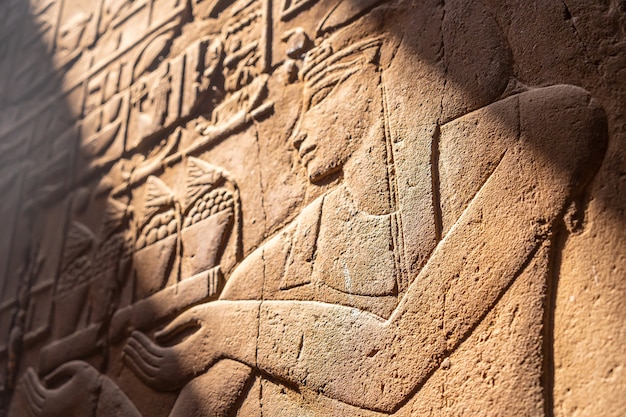The image depicts a detailed terracotta frieze that likely originates from Egypt or an exhibit in a museum dedicated to Egyptian artifacts, possibly the Metropolitan Museum of Art in New York City. The frieze features a realistic and intricate portrayal of what appears to be a significant historical figure, possibly a pharaoh, etched onto a brown stone wall. This central figure is depicted in profile, facing left, with arms turned sideways as if handing something to someone beside him. He exhibits traditional Egyptian features and attire, including characteristic hair. Additionally, there are numerous intricate, almost 3D-like etchings surrounding the central figure, including representations of warriors, baskets of fruit, possibly fish on hooks, and other ambiguous items. A distinct beam of sunlight shines from the top left to the bottom right of the image, further highlighting the detailed carvings and adding depth to the frieze. The sunlight, however, casts shadows that obscure some of the finer details, making specific objects less discernible.